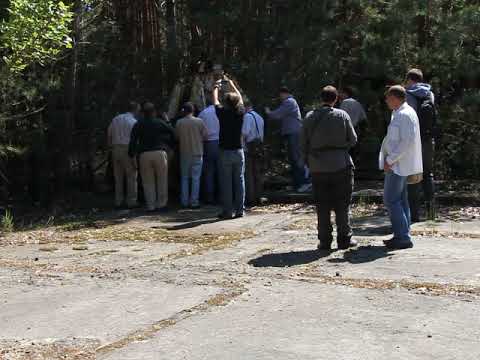In this outdoor image, taken in the middle of the day, we observe a group of roughly twelve men with their backs towards the camera, clustered towards the bottom third of the image. These individuals, who are all wearing long-sleeved shirts and either blue jeans or khaki pants, appear to be somewhat bulky in build. They are holding cameras and are focused on capturing something ahead of them. 

The ground they stand on consists of a concrete or stone pad interspersed with organic debris, such as loose rocks and pebbles, and some vegetation. This stone surface dominates the lower portion of the image, creating a significant negative space. 

Above the men, in the upper left corner and extending towards the upper middle, there is lush vegetation highlighted by daylight, indicating a dense forest or a thick stand of trees. This rich greenery is filled with many tree trunks and dense foliage, allowing minimal sunlight to seep through. The upper right corner also features similar vegetation, emphasizing the natural setting. It appears that this scene could be part of a tourist attraction or a similar outdoor venue where people gather to photograph nature.